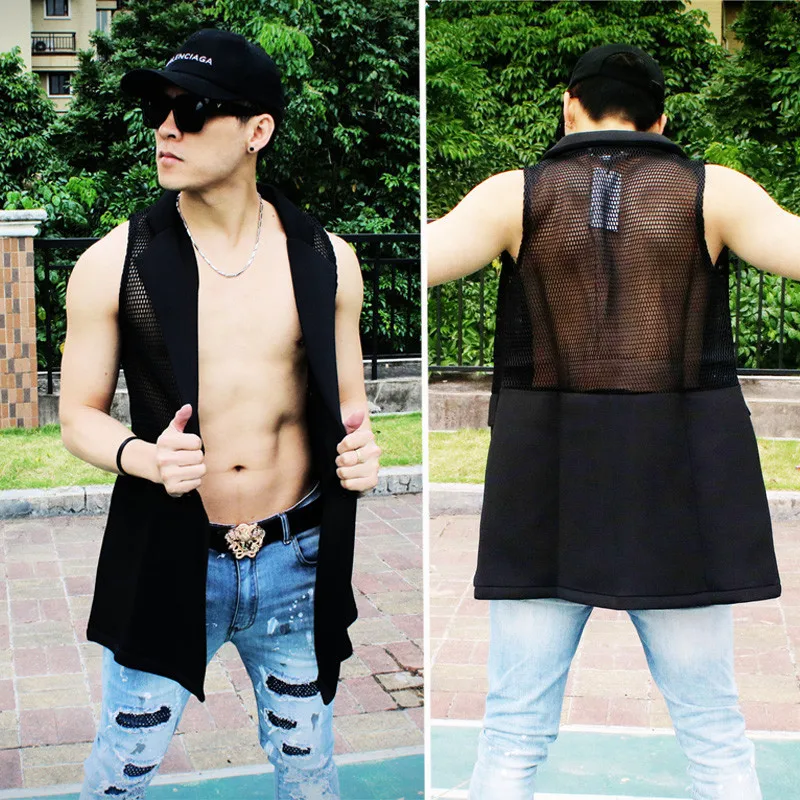The image features a young male model captured from both front and back angles. He is donning a distinctive sleeveless, black mesh vest that leaves his chest, belly, and arms exposed, coupled with black earrings and a black hat adorned with white text. His jeans, which are blue and torn in several places, have been patched with darker blue fabric and are held up by a thick black leather belt with a pronounced brass buckle. The back view reveals the see-through nature of the vest, showcasing his skin beneath the mesh fabric, and highlights his dark hair. The setting is an outdoor brick courtyard, encircled by grass, trees, and apartment buildings, with a metal balcony visible in the backdrop, creating a balanced blend of natural and urban elements.